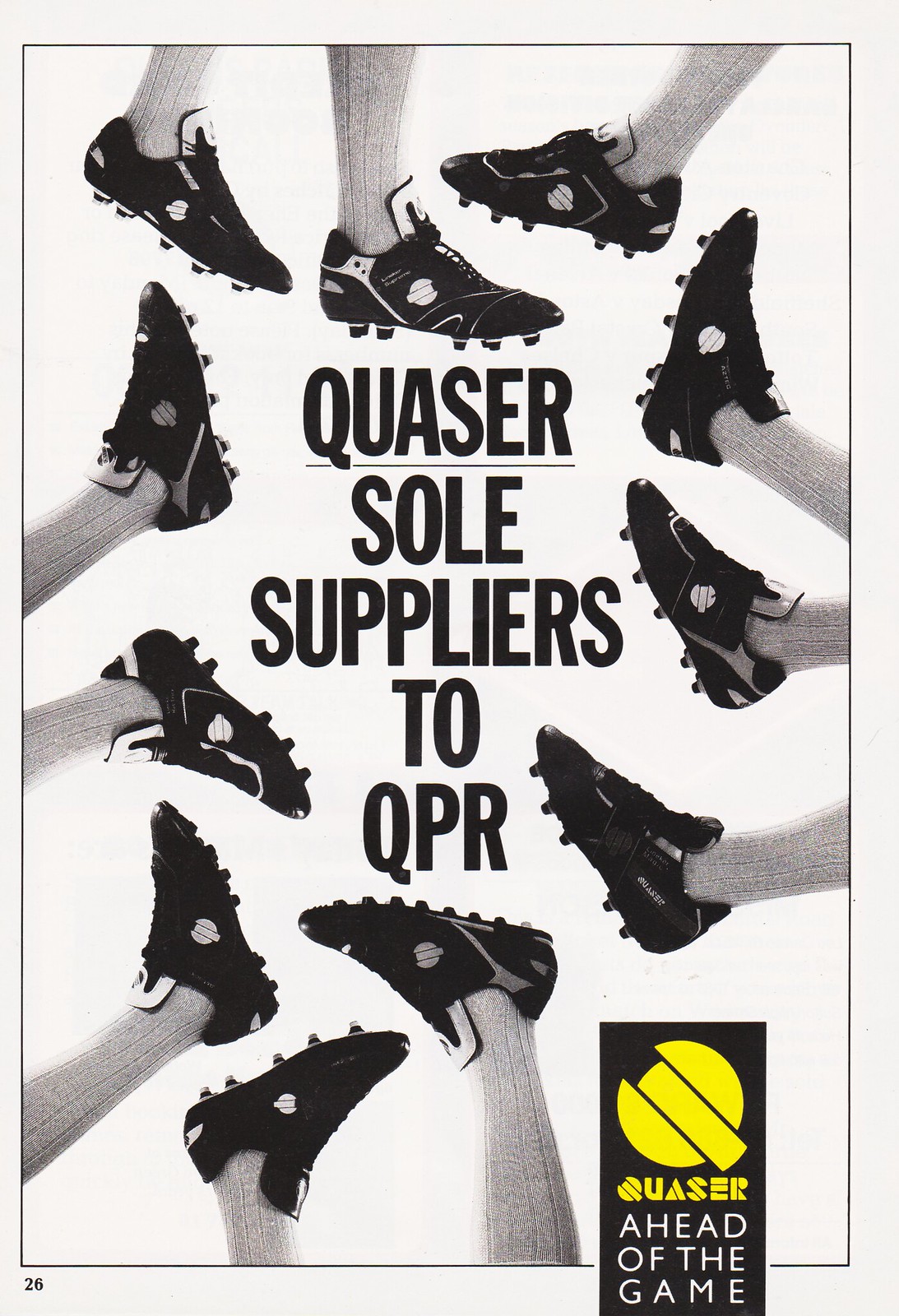The image is a black-and-white advertisement for Quasar soccer cleats, centered around the text, "Quasar sole suppliers to QPR." In the bottom right-hand corner, a black box features a slightly off-center yellow circle with "Quasar" in black letters and "ahead of the game" in white letters. Surrounding the central text are 10 pairs of legs, each wearing shin-high white socks and black soccer cleats with white detailing. The legs radiate outwards in a radial fashion against a light gray background.